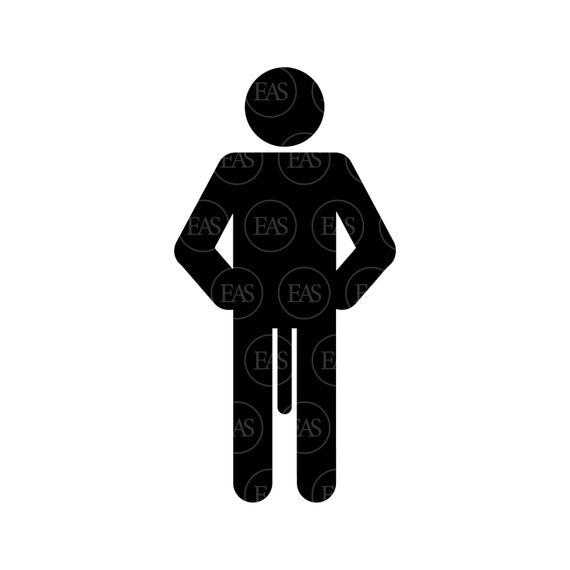The image portrays a solid black, abstract human figure, reminiscent of the generic representations found on restroom doors. The head is a perfect, detached circle, suspended slightly above the torso. The torso is blocky, with thick lines that form the arms and legs. The arms are positioned with the hands resting on the hips; the hands and lower arms are not distinct and appear rounded. The legs are also thick and rounded at the bottom, without visible feet. In between the legs, a long, thin object, resembling either a penis or a tail, hangs down to about knee level. The entire figure features multiple watermarks throughout, consisting of light gray circles with the capitalized letters "E-A-S" inside them. The overall appearance is simplistic yet distinctive, with no facial features and a straightforward, geometric structure.